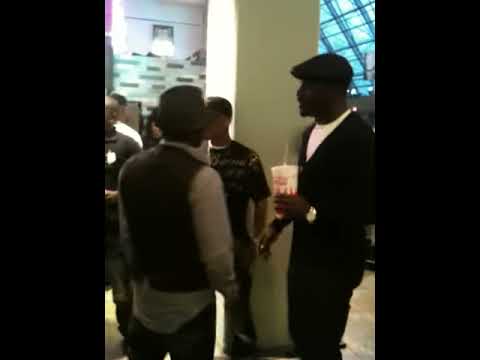In this dark and slightly blurry photo, a group of African American men are gathered, seemingly talking and interacting around a white pillar and wall. The man on the right, the tallest among them, is wearing black pants, a black jacket over a white t-shirt, and a black hat. He is also adorned with a big shiny watch on his left wrist and holds a large soda drink with a straw in his left hand. There is another man with dark pants, a dark vest over a white shirt, and a dark hat, who is facing the tall man. Behind him, resting by the white pillar, is a man in a black shirt with writing on it, with his left hand in his pocket and a watch on his wrist as well. Additionally, there are several indistinguishable individuals in the background, including a man possibly wearing a black collared shirt with a white badge over his chest and another person in a white shirt. The setting includes a window on the right side with light streaming through, a bright ceiling light, and some ambiguous writing on the wall.